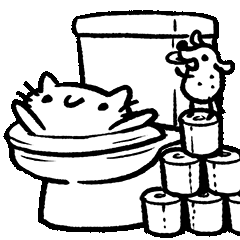This black and white illustration depicts a comically chaotic scene centered on a modern-day toilet. Dominating the left side, the toilet is drawn without a lid and is oriented to face left. A distressed cat, with ears perked and whiskers visible, has its body stuck inside the toilet bowl while its front paws are resting on the toilet seat, and it gazes upwards with a wide-eyed expression. To the right of the toilet, six well-detailed rolls of toilet paper are carefully stacked in a pyramid formation, showing realistic perforated edges. At the apex of this toilet paper tower, a small mouse, illustrated with a dot for a nose, visible eye, flopping ears, and three body dots, stands laughing at the plight of the trapped cat. The mouse's whimsy, accentuated as it reaches toward the toilet's flush handle, adds to the humorous tone of the scene. The clean, thick black lines or perhaps deep black pencil strokes used for the outlines and lighter gray shading give depth and contrast to the meticulously detailed comic-like drawing, which measures approximately two inches by two inches. The overall composition and every intricate element contribute to the whimsical and playful nature, making this a striking, detailed piece of art.